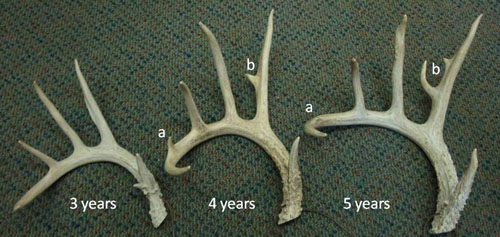This photograph features a clear, overhead view of three sets of deer antlers artistically arranged on a green, textured carpet. The carpet has a thick woven weave with striking hues of grays, blues, and scattered red dots. Each antler set is meticulously positioned in a horizontal row and labeled to indicate the age of the deer at different stages of its life. On the left, the smallest antler, an ivory-ish white in color, curves with three distinct points rising from the apex. Below it, bold white text reads "Three Years." The middle antler is slightly larger and more hooked, showcasing four points – one of which is a small projection near the base – with the label "Four Years" beneath it. Additionally, two points are marked with the letters "A" and "B." The rightmost and largest antler demonstrates a less pronounced curve and more horizontal orientation. It features three prominent spikes and an additional spike branching off the largest point, with "Five Years" inscribed below it. This detailed arrangement highlights the progressive growth of antlers over the years.